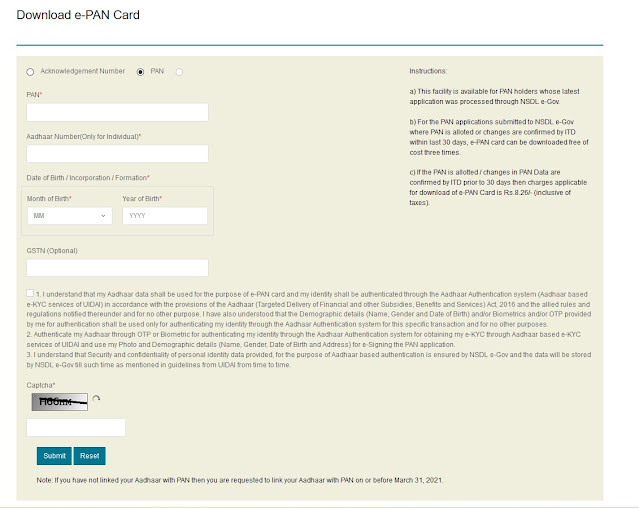The image depicts a low-resolution screenshot of a website's data entry page. The page has an off-yellow background adorned with black printed text. In the upper right corner, there are instructions labeled "A, B, C," though the exact details remain unreadable due to the blurriness. On the top left, the page features options with radio checkboxes—small white circles—where users can select one of the provided choices. There are three radio circles but only two associated statements. The leftmost option is labeled "Acknowledgment Number," while the option to its right, marked with capital letters, is "PAN," which appears to be the selected option. An additional blank radio selection follows.

Directly below these choices, a white text entry line is positioned under the "PAN" label. Further down, there's a field for "AADHAAR Number" specifically for individuals, followed by a text entry box. Below this entry, users can input their "Date of Birth" or "Corporation Formation" details, with options for the month and year of birth. The subsequent section offers a text entry line for "CSTN" (optional).

At the bottom of the form, there's an incomplete, illegible checkbox statement emphasizing that "AADHAAR data will be used for" an unspecified purpose. Finally, the page provides two blue buttons with white lettering: "Reset" and "Submit."